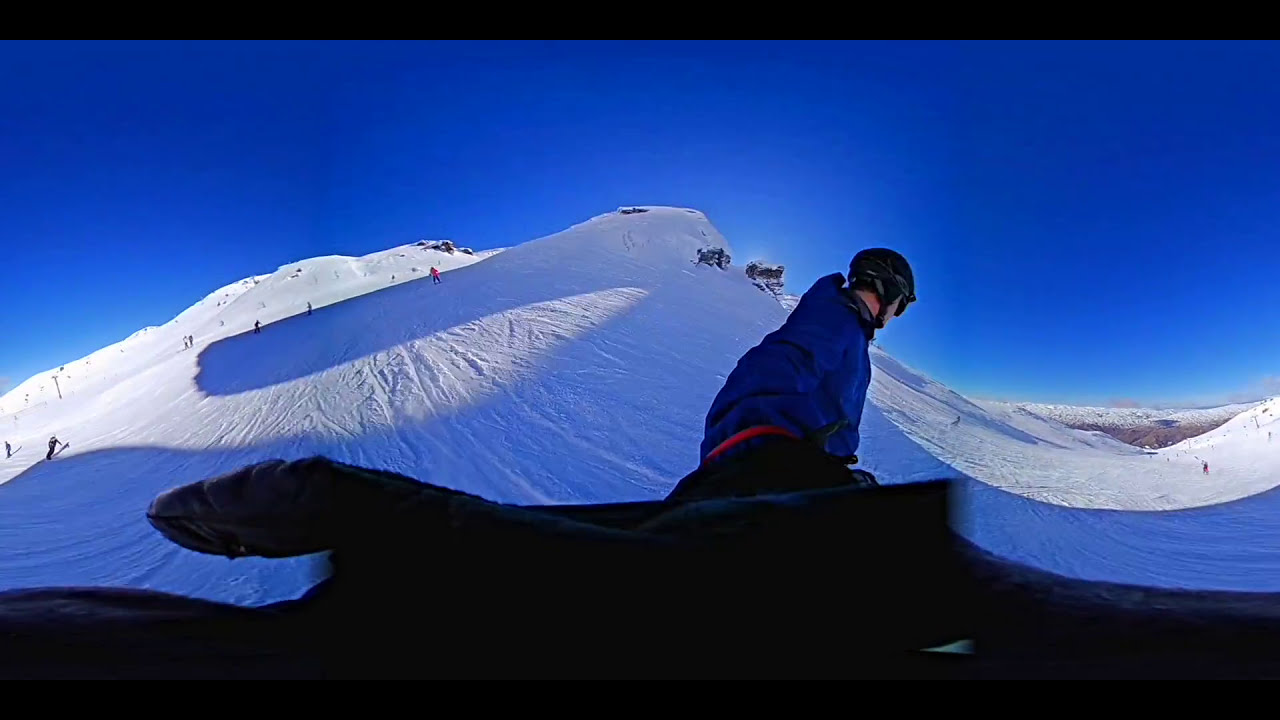This captivating image captures the exhilarating moment of a man snowboarding down a steep, snow-covered mountain, as seen through his selfie stick. The snowboarder, positioned centrally near the bottom of the frame, is outfitted in a blue snow jacket, black safety helmet, black goggles, and black pants, indicating his readiness for the cold, outdoor adventure at what appears to be a bustling ski resort. Behind him, the image showcases around ten fellow skiers and snowboarders descending the slope, while a couple more can be spotted ahead of him. The rugged, jagged peak of the mountain protrudes through the snow in the background, encapsulating the essence of an alpine setting under a clear, vibrant blue sky. The wide angle shot also reveals a sweeping view of the terrain, exaggerating the vastness of the snow-covered slope and emphasizing the thrill of the descent.